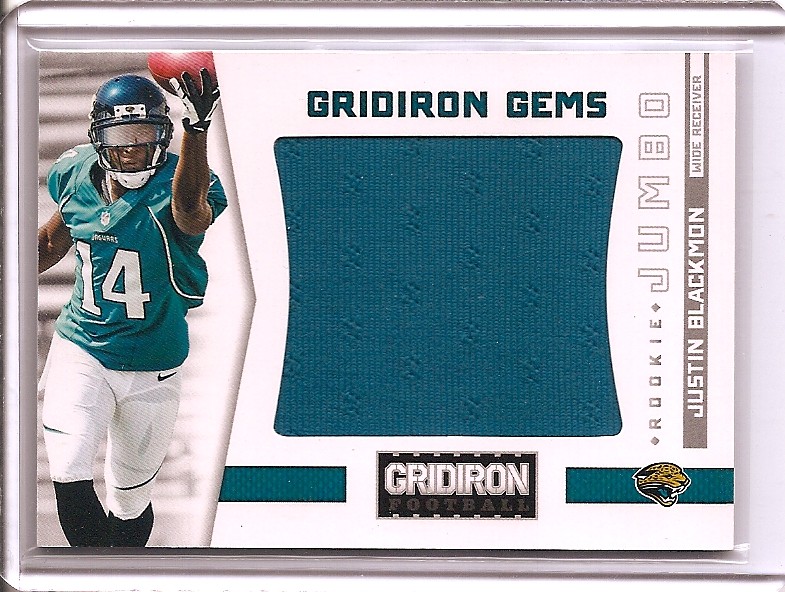The image displays a detailed scanned copy of a football card inside a protective top loader and clear plastic sleeve. The left side of the card features a photograph of Justin Blackman, a member of the Jacksonville Jaguars, identifiable by his dark green jersey with the number 14, paired with white football tights and black socks. He is also wearing a green helmet and white and black gloves while holding a football in his left hand. The background of the card is predominantly white, with silver borders. 

The text elements on the right-hand side include "Gridiron Gems" in dark blue at the top, and directly below it, a transparent segment showcasing a fabric patch from his jersey. Further down, "Gridiron Football" is inscribed in white font inside a black box. Along the right edge of the card, the words "Rookie Jumbo" are placed vertically in silver font. At the bottom, within a light gray box, "Justin Blackman" and "Y Receiver" can be seen clearly in white text.